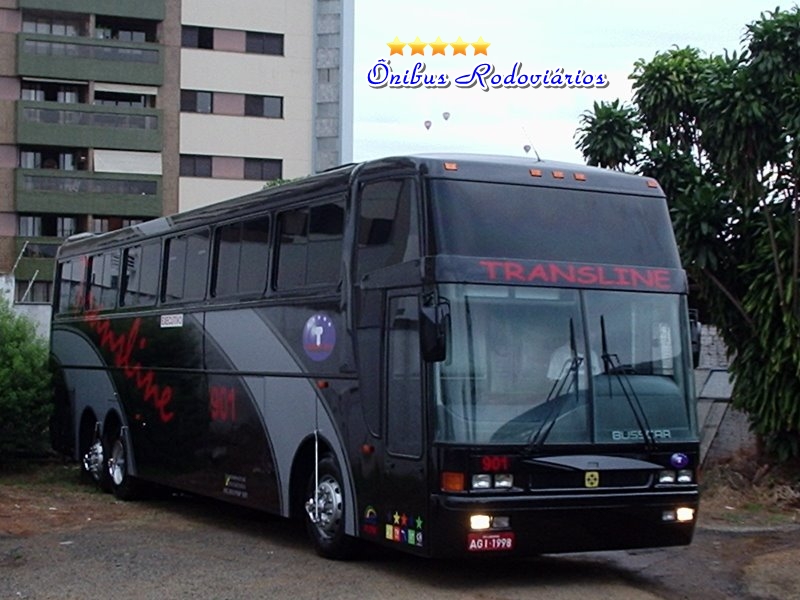The image depicts a sleek, black city bus parked in a semi-urban parking lot. Prominently displayed on the front of the bus, above the driver's seat window, is the red text "Transline." Additionally, "Transline" is printed on the side of the bus. A digital display and tinted windows are also visible, with the driver seen through the large front window wearing a white t-shirt. The bus has several sets of double windows positioned high, indicating a raised passenger area accessible by stairs. 

A watermark featuring five yellow stars and the text "Onibus Rodoviarios" in blue is placed above the bus in the image. The background reveals a towering apartment building complex with a whitish-tan facade that reaches up to six stories high. Surrounding the parking lot are bushes and trees, adding to the semi-urban feel of the scene. A red license plate marked "AGI 1998" is on the left side of the bus, which is illuminated by lights on its front bumper. The overall setting combines urban and natural elements, capturing a moment that could easily serve as an advertisement or a postcard for luxury travel.